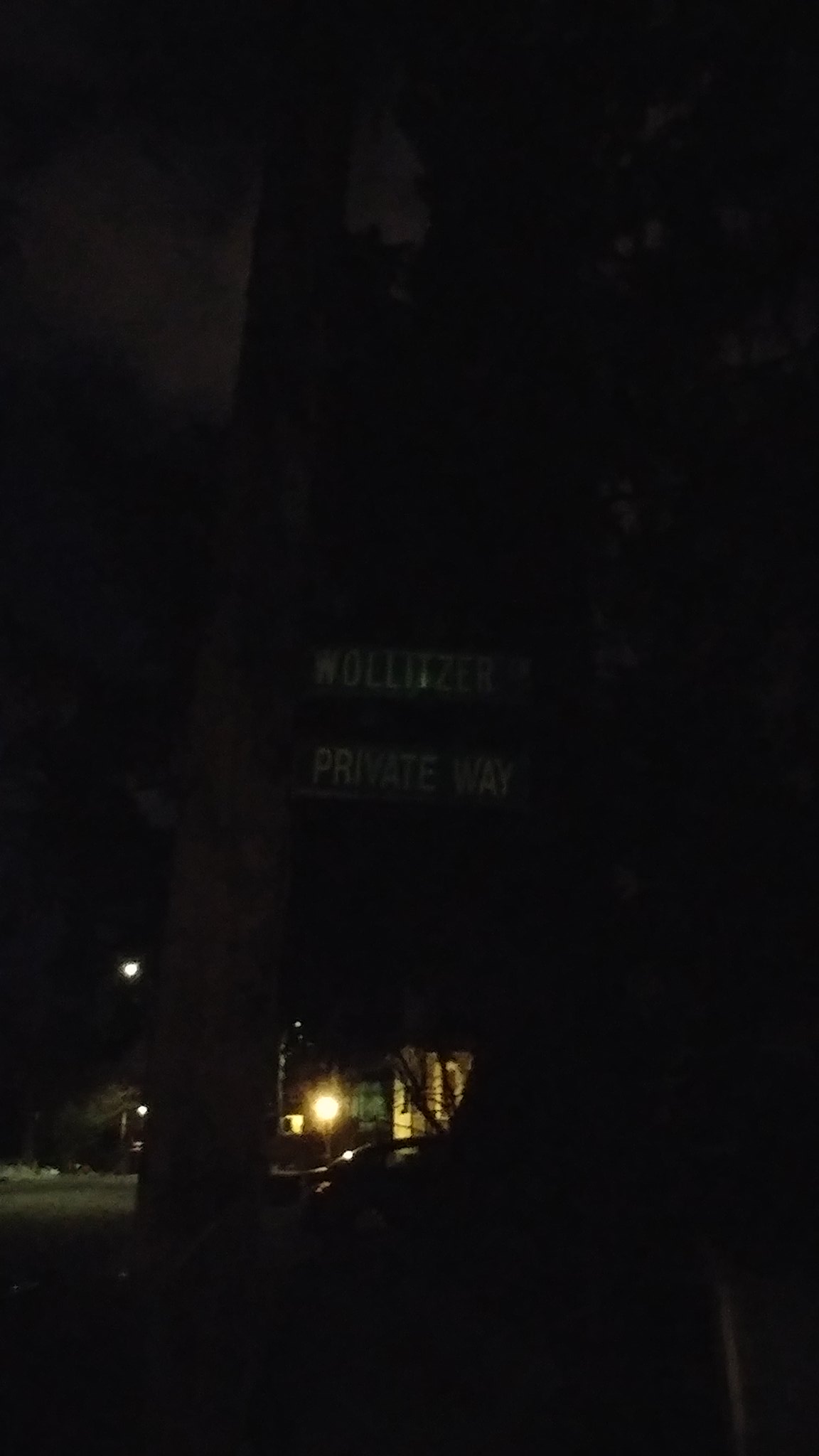In this nighttime photograph, taken outdoors on a street, the focal point is a street sign prominently displayed in the foreground. The sign reads "Wollitzer Private Way," with the letters clearly visible despite the low light. It hangs above head height, requiring the camera to be angled upward. The background reveals muted street lights and porch lights, casting a faint glow around the scene. An automobile is faintly outlined in front of a residential house. The sky is predominantly dark, but a grayish hue behind a tree line hints at the presence of moonlight, adding a subtle atmospheric touch to the image.